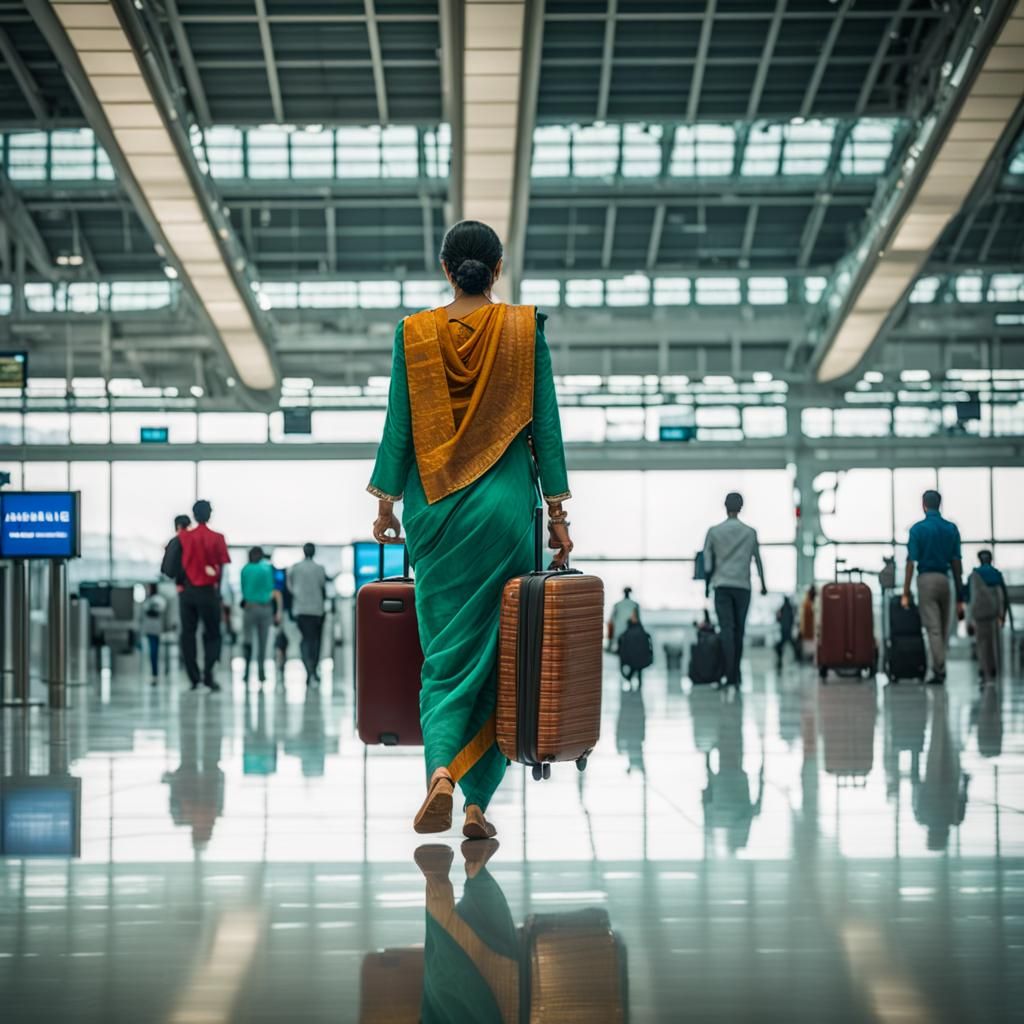A woman walks away from the camera in an airport, holding an orange hard-shell suitcase in her right hand. The suitcase stands out against the bustling airport environment. The camera angle is slightly tilted upwards, capturing both the ceiling and the floor, and providing a sense of the airport's spacious interior. Other travelers can be seen in the background, also walking in the same direction, some with their own luggage in tow. A blue directional sign is visible to the left, hinting at the organized flow of the terminal. The image is a close-up, focusing on the woman and her vibrant suitcase, yet it captures the essence of the busy airport scene around her.